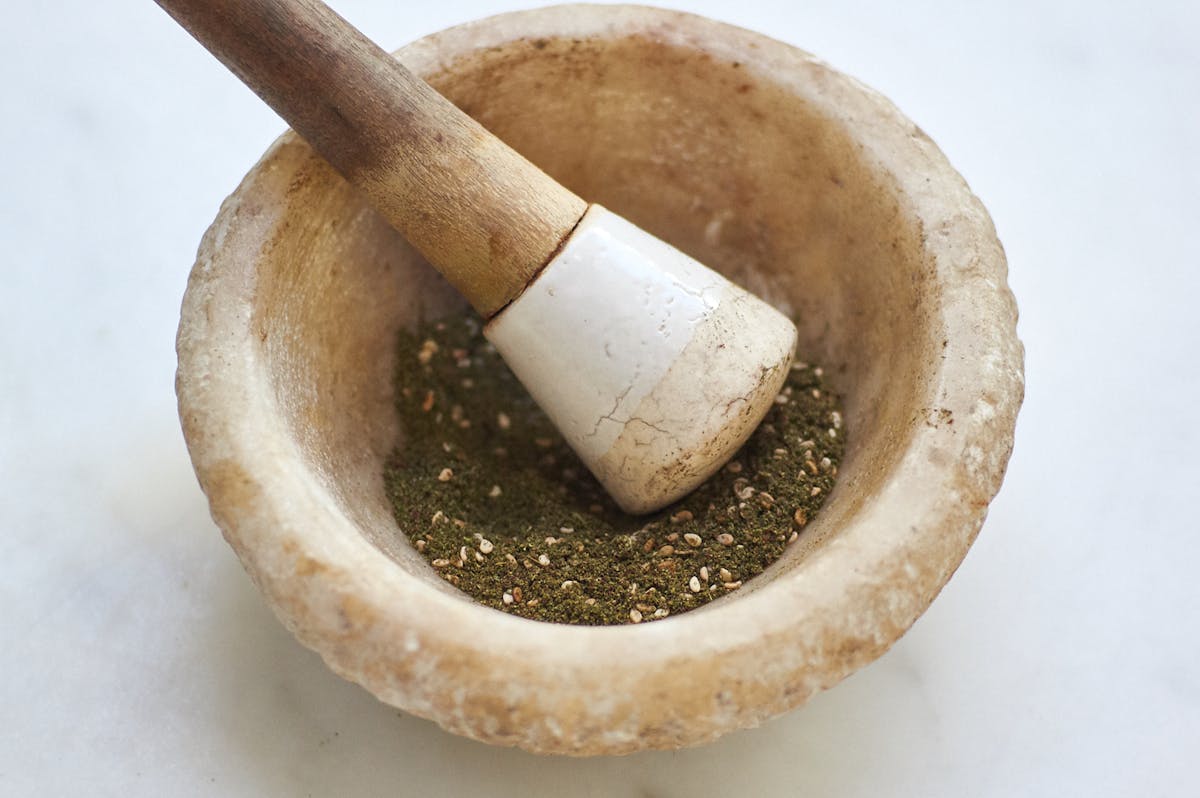In this image, a ceramic mortar and a wooden-colored pestle are seen on a white surface. The interior of the bowl features finely ground ingredients, possibly spices, with the pestle actively grinding them. The setting is minimalistic, focusing solely on the mortar and pestle, emphasizing the meticulous grinding process taking place.